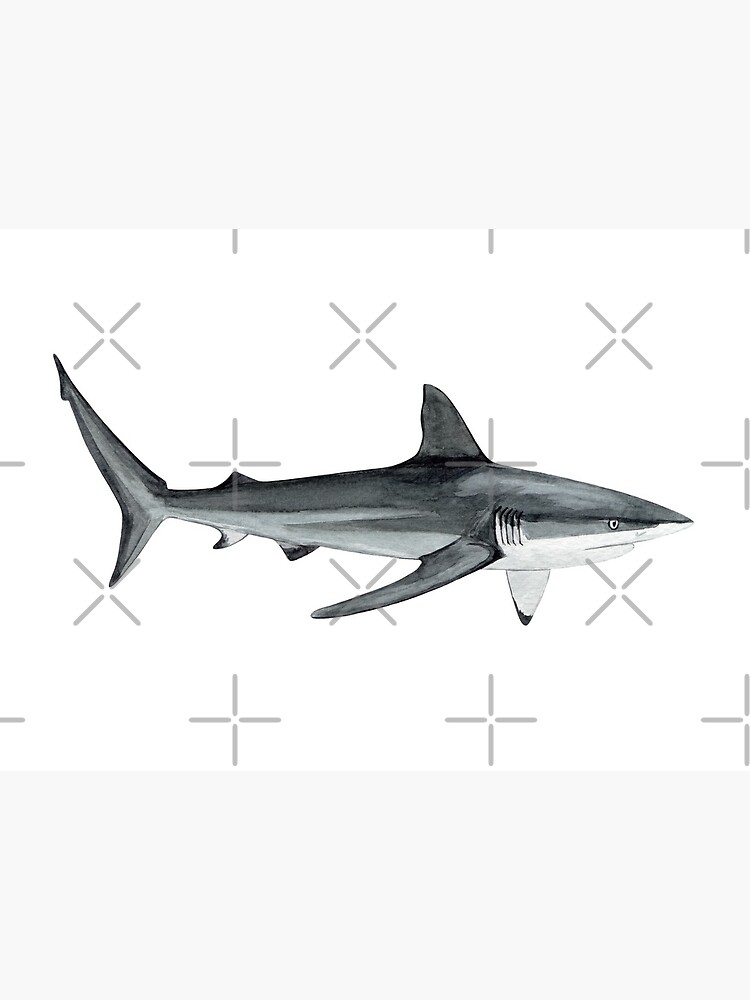This is a dark, ominous illustration of a tiger shark rendered in ink or watercolor on a stark white background. The right side of the shark is prominently displayed, with its pointed fins and large dorsal fin vividly depicted. The shark's color transitions from a dark gray on top to lighter shades, including whites and light grays, on the bottom half, starting from the snout and extending backward. Its eyes, intense and seemingly angry, add to the menacing aura of the creature. Over the shark's body, there's a watermark or text in white, uppercase letters, spelling out "BEATRIZ ABAITUA." No other objects interrupt the minimalist composition, focusing all attention on the formidable presence of the shark.